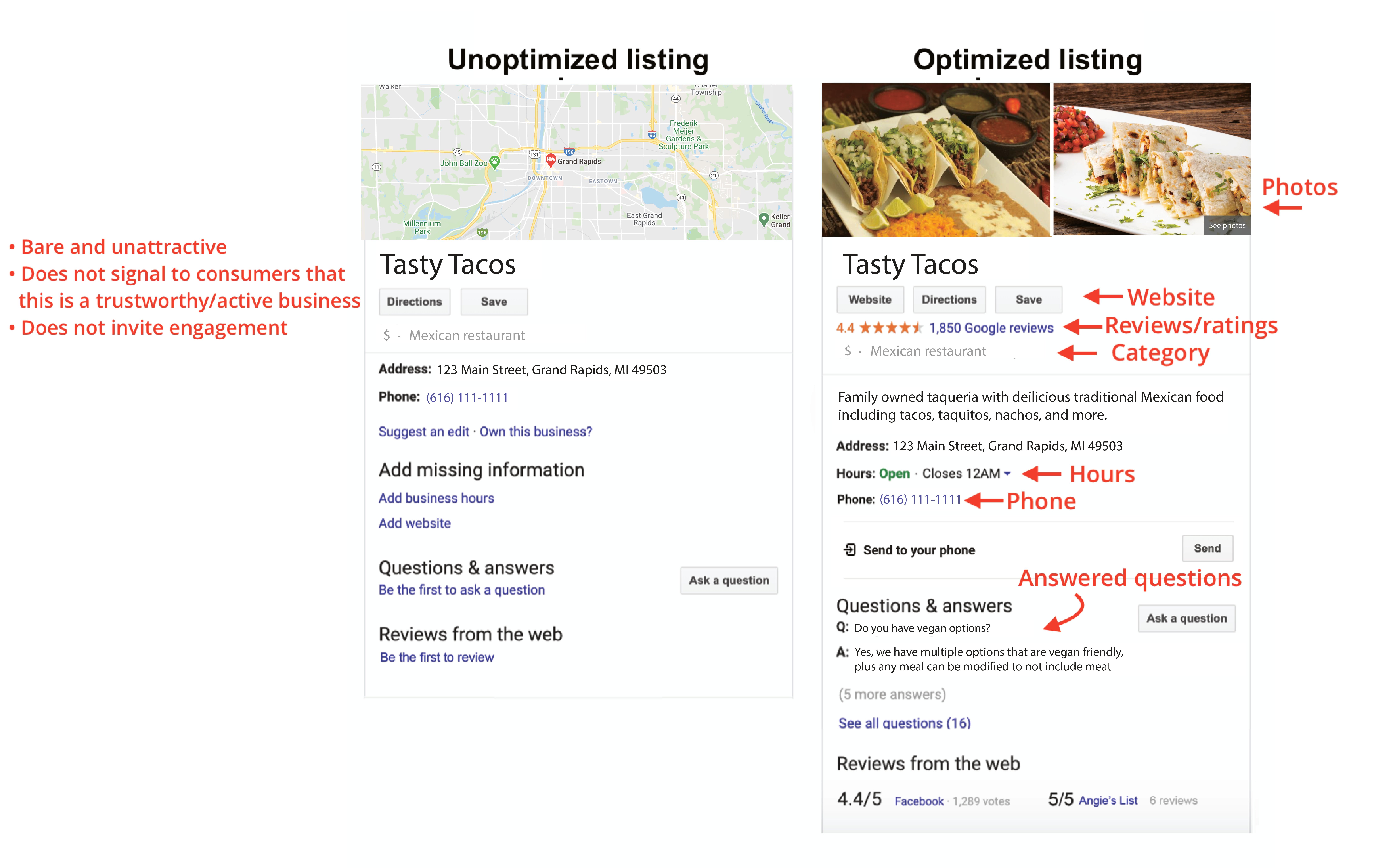This webpage provides a detailed overview of Tasty Tacos, combining elements from Google Maps and their own site to suggest ways to optimize their listing for better engagement.

**Webpage Overview:**

**Left Section:**
- **Red Text Annotations:**
  - "Bare and unattractive"
  - "Does not signal to customers that this is a trustworthy/active business"
  - "Does not invite engagement"

**Center Section:**
- **Map Section:**
  - Title: "Unoptimized listing"
  - Below the Map: "Tasty Tacos"

**Details Below Map:**
  - **Category:** Mexican Restaurant
  - **Buttons:** 
    - Directions (mid-gray with black text)
    - Save
  - **Address:** 
    - "123 Main Street, Grand Rapids, MI 49503" (bold)
  - **Phone:** 
    - "(616) 111-1111" (bold, blue text)
  - **Editable Options:** 
    - "Suggest an edit"
    - "Own this business?"
  - **Additional Info:**
    - "Add missing information"
  - **Clickable Options:**
    - "Add business hours"
    - "Add website"
  - **Questions and Answers:**
    - "Be the first to ask a question" (blue, clickable)
    - "Ask a question" button (mid-gray with black text)

**Reviews Section:**
  - **Title:** "Reviews from the web" (bold)
  - "Be the first to review" (blue, clickable)

**Right Section:**
  - **Photos of Tacos:**
    - Yellowish tortillas with orange lettuce, brown beef, and cheeses including cheddar and possible Monterey Jack.
    - Accompanied by dipping sauces: deep red, light red, and green chili sauce.
    - Close-up of soft tacos with green garnish, flavored orange chicken, diced tomatoes, and purple onions on a white platter.
  - **Clickable Options:**
    - Website (mid-grade, black text)
    - Directions
    - Save
  - **Red Text Annotations:**
    - "Photos" suggesting the inclusion of photos for better optimization.
    - "Website" pointing towards the website link.
    - "Reviews/ratings: 4.4/5 stars from 1,850 Google Reviews" (orange stars, 1,850 hyperlinked in blue).
    - "$" indicating affordability.
    - "Category: Mexican Restaurant" with a red arrow suggesting selecting appropriate categories.

**Additional Information Panel:**
  - "Family-Owned Tequila Taqueria with delicious traditional Mexican food including tacos, taquitos, nachos, and more."
  - Repeated address: "123 Main Street, Grand Rapids, MI 49503"
  - **Opening Hours:**
    - Bold green text: "Open" and "Closes 12 a.m." with a drop-down arrow.
  - **Phone Number Reiterated:**
    - "(616) 111-1111" with red arrow highlighting the phone number.
    - "Send to your phone" option with send button (mid-gray, black text).

**Questions and Answers Panel:**
  - **Example Question:** "Do you have vegan options?"
    - **Answer:** "Yes, we have multiple vegan-friendly options and meals can be modified to exclude meat."
  - **Red Text Annotations:** "Answer Questions" suggesting the business should engage with customer inquiries.

**Review Summary from Other Platforms:**
  - Facebook: 4.4/5 based on 1,287 votes (clickable in blue).
  - Angie's List: 5/5 based on 6 reviews (gray text).

This detailed webpage aims to improve Tasty Tacos' online visibility by providing comprehensive information, customer engagement options, and clear calls to action for both potential customers and the business owner.